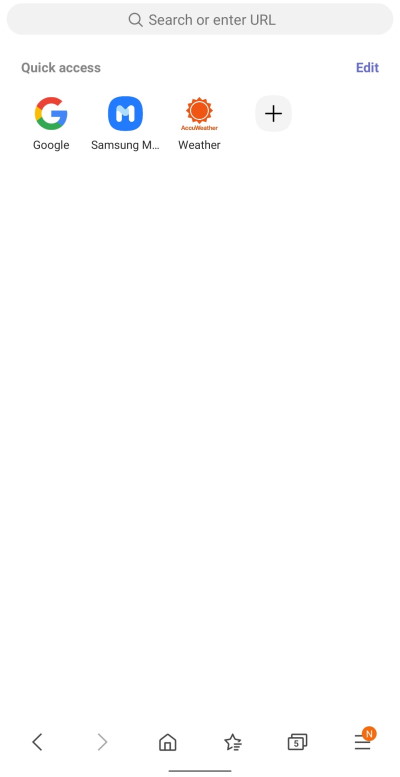The image depicts a user interface layout, likely of a browser's start or home page. At the very top, there is a gray area featuring a magnifying glass icon next to the text "Search or enter URL." Below this, aligned to the left, the text "Quick Access" is displayed, and to the right of this text is a blue hyperlink labeled "Edit." 

Under the "Quick Access" section, the first item on the left showcases the multicolored Google "G" logo, with the word "Google" written underneath it. To the right of this, there's a blue box with a white "M" in its center, labeled "Samsung M" below. Further to the right, an icon displays an image of a sun rising into the sky, labeled "Weather."

Adjacent to the "Weather" icon, there is a gray box with a plus symbol in the middle. Below these icons, the background is plain white, void of any content. Finally, at the very bottom of the interface, there are several navigation symbols including a less than symbol ("<"), a greater than symbol (">"), a home icon, a favorites icon (star), and a hamburger menu button, which has an orange box at its top.